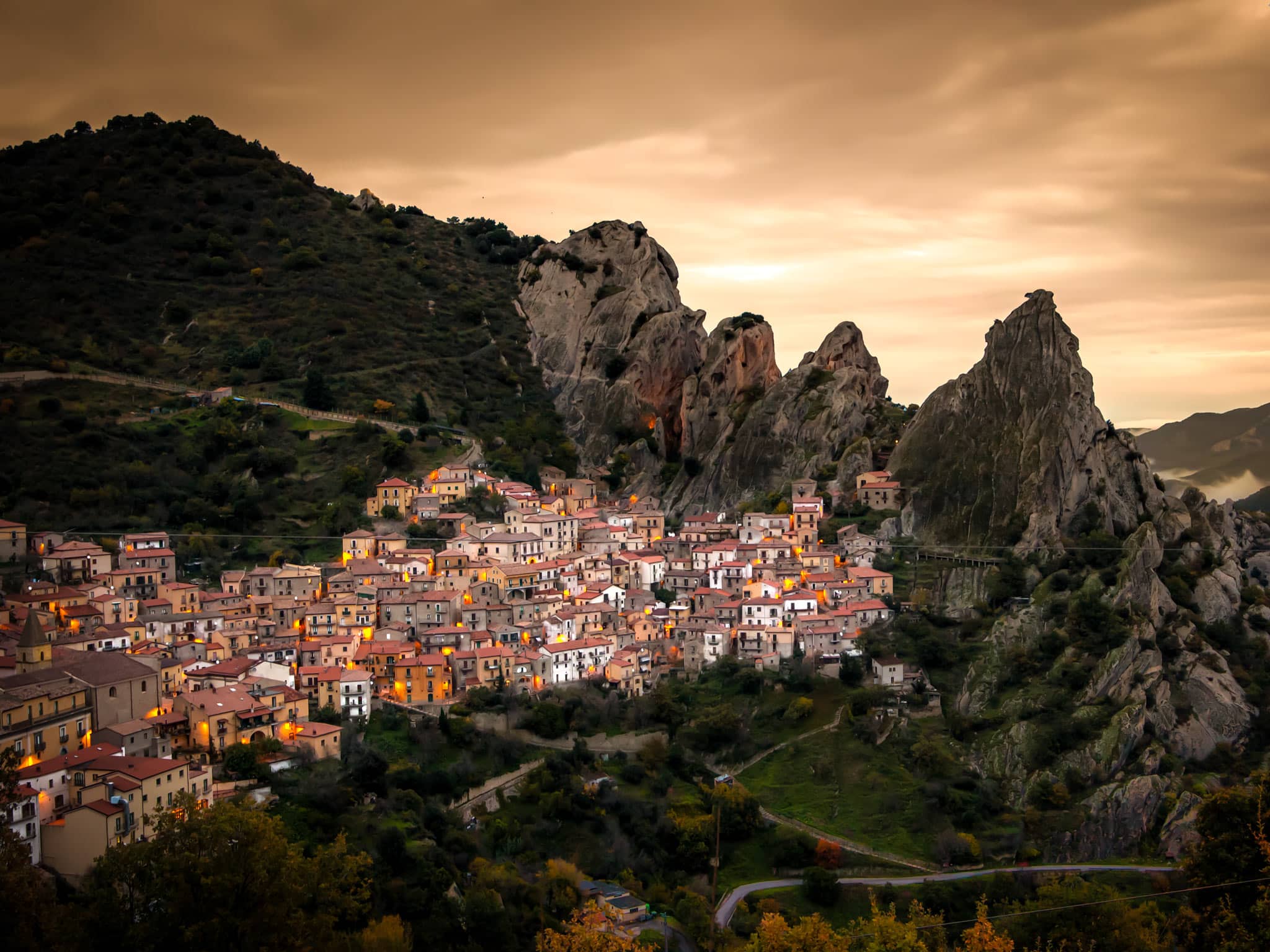This photograph captures a quaint, charming village nestled in a lush green valley surrounded by craggy mountain peaks. The village is composed of tightly-packed two and three-story buildings featuring red and brown roofs, with white plaster or stucco walls. The landscape is dotted with narrow, gray roads winding through the green foliage, adding to the picturesque scenery. The shot appears to be taken from a high vantage point, likely from a drone or helicopter, offering a clear view of the valley and the mountains. To the left and center of the image, steep rocky cliffs stand tall, while to the right, the horizon stretches into the distance under a cloudy, overcast sky tinged with red streaks from the setting sun. The atmospheric lighting creates a warm, inviting feel, enhanced by the soft yellow-orange lights glowing from the exteriors of the village homes, making it look like an idyllic, serene place for a peaceful vacation.